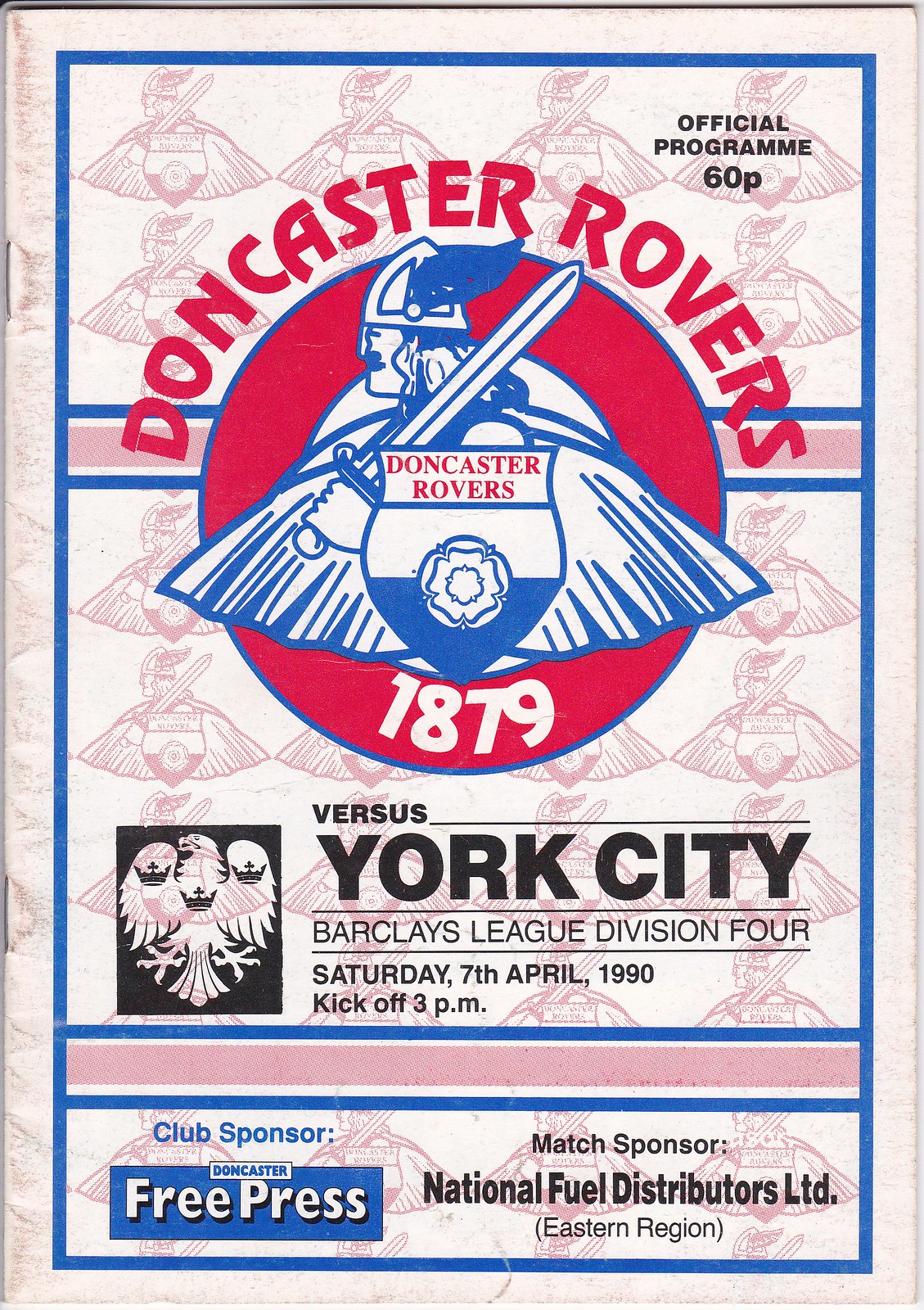This detailed and composite caption describes an official program cover for a Doncaster Rovers football match against York City, held on Saturday, April 7, 1990, at 3 p.m. The program, priced at 60 pence, has a white background with numerous red Doncaster Rovers logos scattered throughout, bordered by a blue frame. In the top right-hand corner, in black lettering, it reads "Official Program 60P." Dominating the center is the prominent Doncaster Rovers emblem, featuring a Viking holding a sword and shield, both depicted in a blue outline filled with red. The shield bears the name "Doncaster Rovers," along with the year "1879," which signifies the club's founding year. Below the main logo, in black text, are the match details: "Versus York City, Barclays League Division 4, Saturday, 7th April 1990, kickoff, 3 p.m." At the bottom, further details mention the club's sponsor, "Doncaster Free Press," in blue, and the match sponsor, "National Fuel Distributors Limited, Eastern Region," in black.